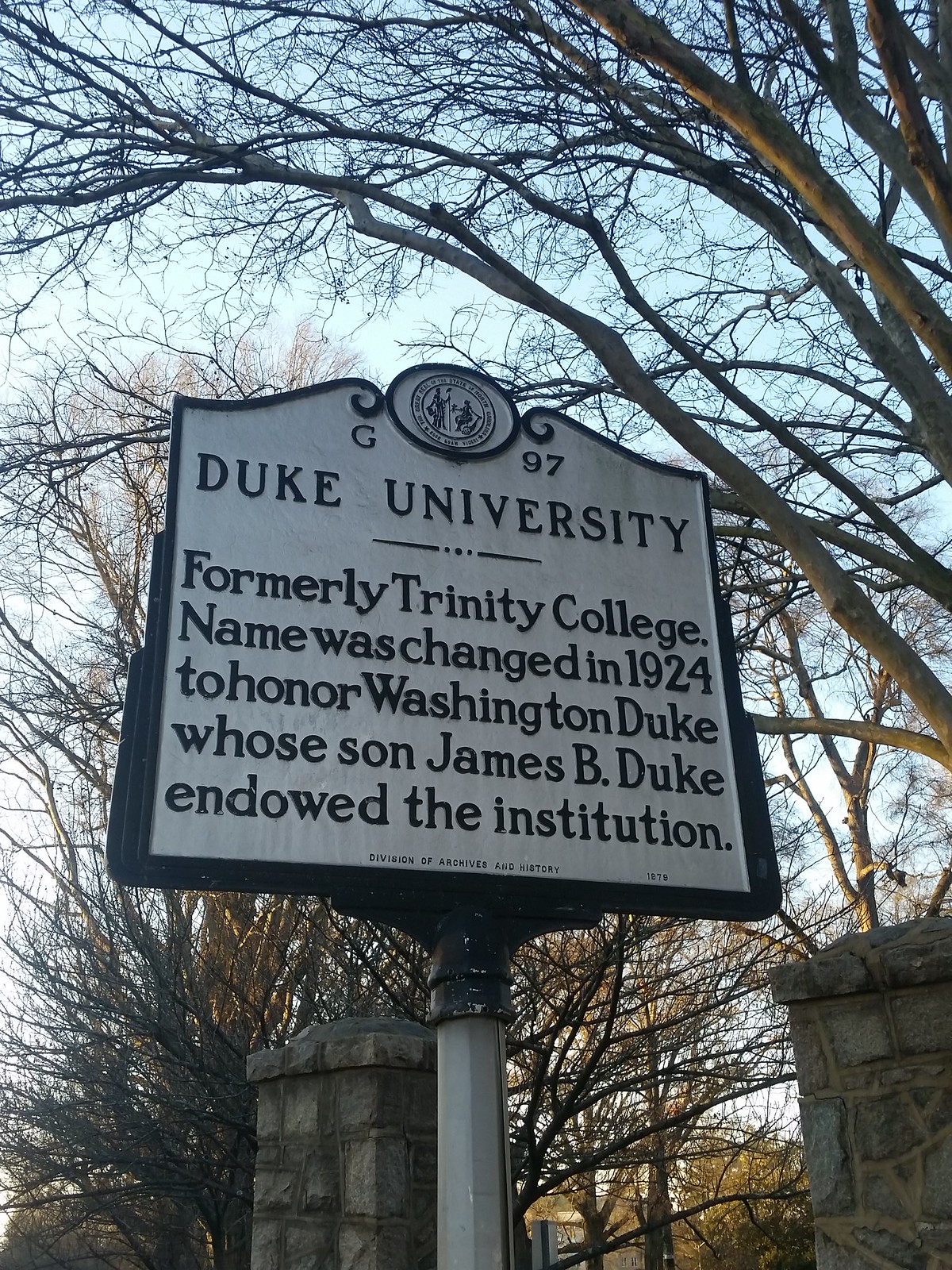This photograph captures an ornate sign on a university campus displaying the text "G97" next to an indiscernible logo, and reading "DUKE UNIVERSITY" in bold black letters, followed by "formerly Trinity College. Name was changed in 1924 to honor Washington Duke, whose son, James B. Duke, endowed the institution." At the very bottom, it states in small text "Division of Archives and History, 1879." The sign, outlined by a black border with a white center, features rounded corners and is mounted on a white pole. Surrounding the sign are two substantial stone columns and a backdrop of trees and vegetation, suggesting a chilly winter day. The lighting hints at either early morning or late evening due to the dimness and the sign being in the shade. The sky appears a clear blue, contributing to the peaceful and historical ambiance of the scene.